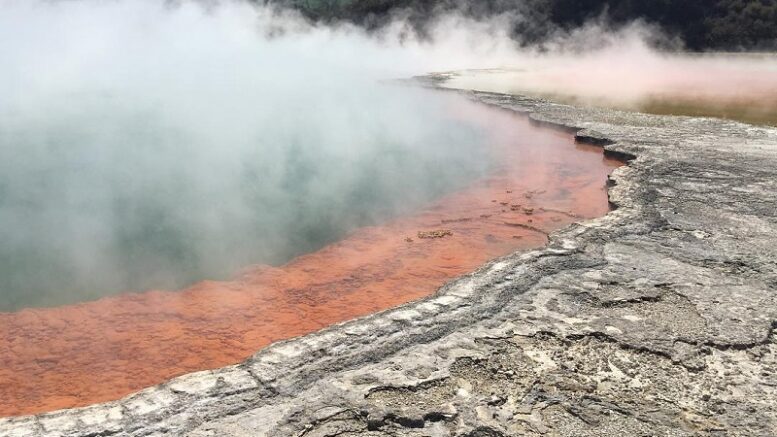The image depicts a natural hot spring characterized by a circular body of water surrounded by gray, wavy, and crumbling rock formations. Steam and fog rise intensely from the water's surface, obscuring much of the view. The pathway leading to the hot spring curves to the right and is cracked and worn, indicating it formed naturally. At the water's edge, there's a slight drop-off from the pathway into the shallowest part of the spring, where copper-colored sand is visible. This sandy area transitions abruptly into deeper, darker water, from which thick steam emanates. The left side of the image is notable for the dense smoke rising from the hot spring, shrouding the scene in a mysterious, ethereal fog.